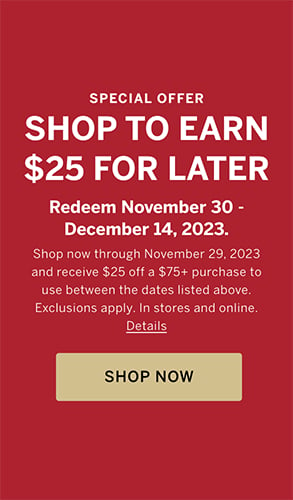The image is a web banner advertisement, featuring a vertical rectangle with a vibrant deep red background. At the top center, the text "SPECIAL OFFER" is prominently displayed in bold, white, all-capital letters. Beneath this, in even larger all-capital white letters, the text reads "SHOP TO EARN." Adjacent to this, there's a dollar sign followed by "$25 FOR LATER."

Below this main message, there's smaller but still significant text with the first letter of each word capitalized. It states, "Redeem November 30 - December 14, 2023." Further down, in finer, lighter print, the details specify, "Shop now through November 29, 2023, and receive $25 off a $75+ purchase to use between the dates listed above. Exclusions apply in stores and online." The word "Details" is emphasized with a capital D and underlined.

At the bottom of the advertisement, there's a golden button in a soft metallic Las Vegas gold color. This button features the text "SHOP NOW" in bold, black, all-capital letters.